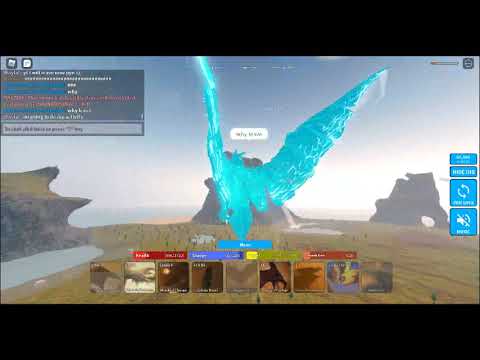The image is a screen from a video game, with long black bars at the top and bottom of the image. The game features an animated, desert-like terrain with a blue sky. The central focus of the image is a massive, turquoise dragon or bird-like creature with a gigantic wingspan, seemingly made of energy or water, flying over the vast landscape towards three large rock formations. In the upper left-hand corner of the screen, there is a gray conversation bar with undecipherable blue, white, and coral text. Across the bottom of the screen, there are approximately nine small squares, each depicting different desert scenes, likely representing different players in a multiplayer gaming platform. The scene conveys a sense of a dystopian or otherworldly environment, enhanced by the bird-like creature's ethereal presence.